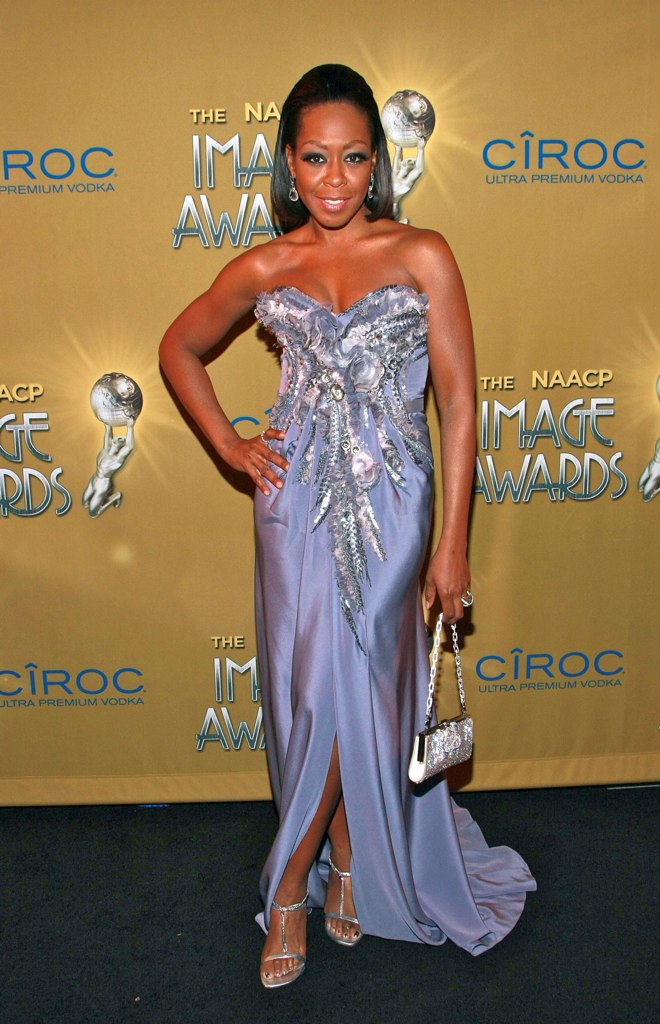In this vibrant image from the NAACP Image Awards, an elegantly dressed African American actress stands poised against a golden and brown backdrop that prominently features logos for Ciroc Ultra Premium Vodka and the Image Awards. She is known for her role in a 90s sitcom, likely evoking nostalgia for shows like "Family Matters." Her sleek black hair is styled back, drawing attention to her bright smile and bluish eye shadow that perfectly complements her dark skin and lean, muscular arms and shoulders. The actress radiates glamour in a strapless purple gown adorned with intricate silver floral designs on the bodice, cascading into a shiny, lavender-gray flowing skirt. She accessorizes with a small, silvery purse held in one hand, multiple rings, and strappy silver high-heeled shoes that reveal her toes. Posing confidently with one foot in front of the other and one hand resting on her waist, she perfectly embodies the grace and sophistication befitting the esteemed event.